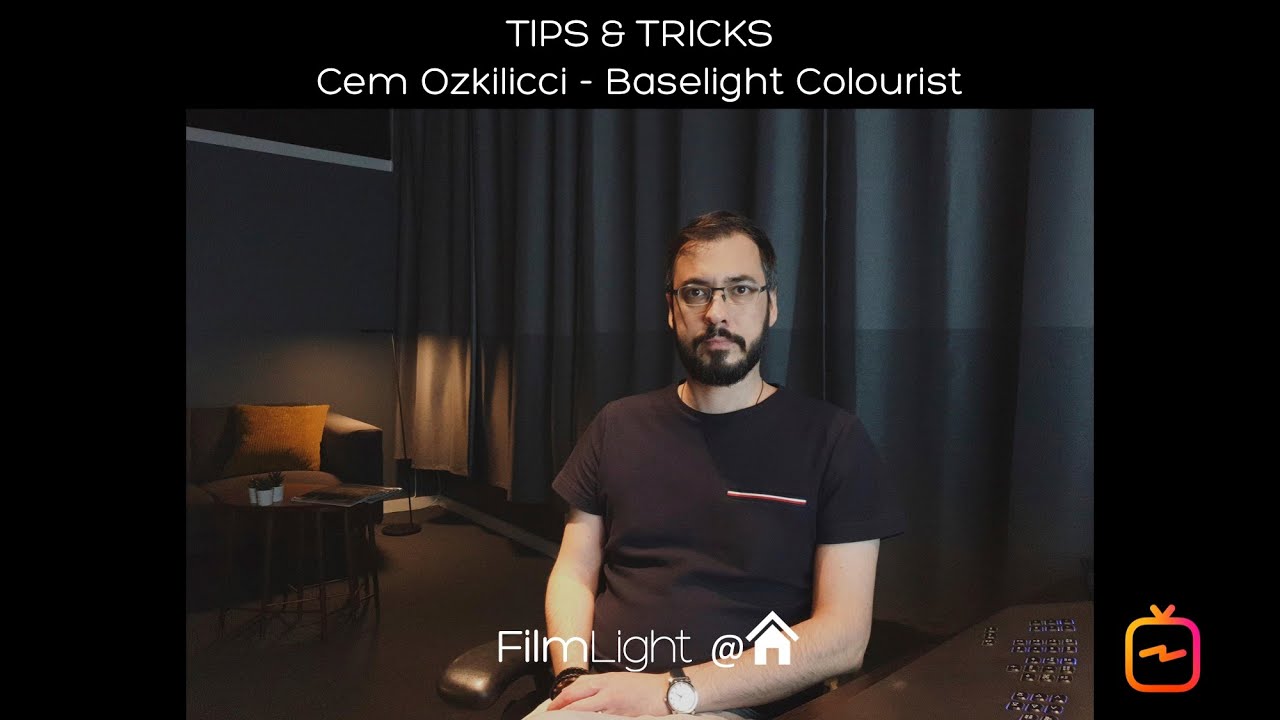This is a detailed photo capturing a bearded man with short brown hair and fair skin, seated in an office or studio setting. He wears frameless glasses and a black short-sleeve shirt, with a large analog watch on his left wrist and his hands resting in his lap. The man stares directly into the camera, displaying a neutral expression. The room is dimly lit, suggesting a nighttime ambiance, and is backed by a large gray curtain.

In the background, on the left side of the image, is a couch partially visible with a brown pillow on it, near which stands a floor lamp subtly illuminating the area. An end table or control board next to the couch holds a few cups, adding to the studio's cluttered but cozy feel. The man is seated in an office chair, with a bit of furniture and a lighted corner forming the backdrop to his right.

Overlaying the center of the photo are the words "Film Light," with a house logo, while at the top, "Tips and Tricks" is prominently displayed in white letters. Below, the text reads "Film Oscillacy - Baselight Colors." The entire picture is bordered by a thick black frame, which does not cover the bottom edge. In the bottom right corner, there is a logo depicting a TV with a zigzag in the center.